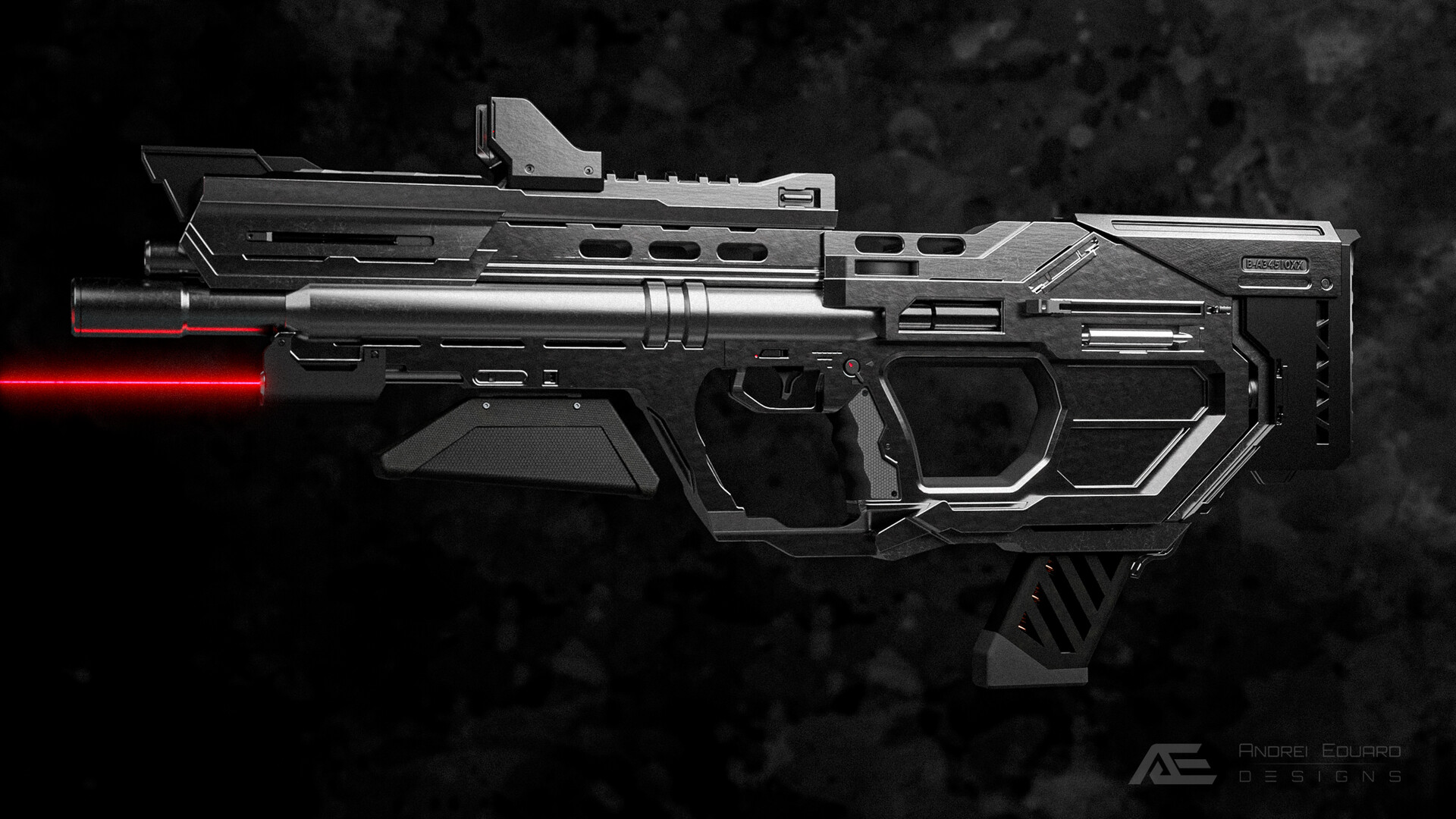This color photograph, created by Andrea Eakward Designs, features a futuristic, computer-generated handgun prominently displayed against a black, gray, and white camouflage background. The weapon itself is sleek and complex, predominantly black and gunmetal gray, with some silver detailing. The barrel is extended towards the left side of the image, and a red laser beam emanates from a laser scope attached beneath it. A notable design feature includes a small handle with an adjacent stock that appears unextended, as well as a top-mounted scope aligned with five ovular holes beneath it. The gun also includes two handle brackets around the trigger area. The intricate nature and high-tech appearance of the firearm give it a uniquely futuristic and perhaps somewhat "Tron-like" feel. In the bottom right corner, the stylized AE logo, representing Andrea Eakward Designs, is visible, slightly transparent, and blending seamlessly with the camo background.